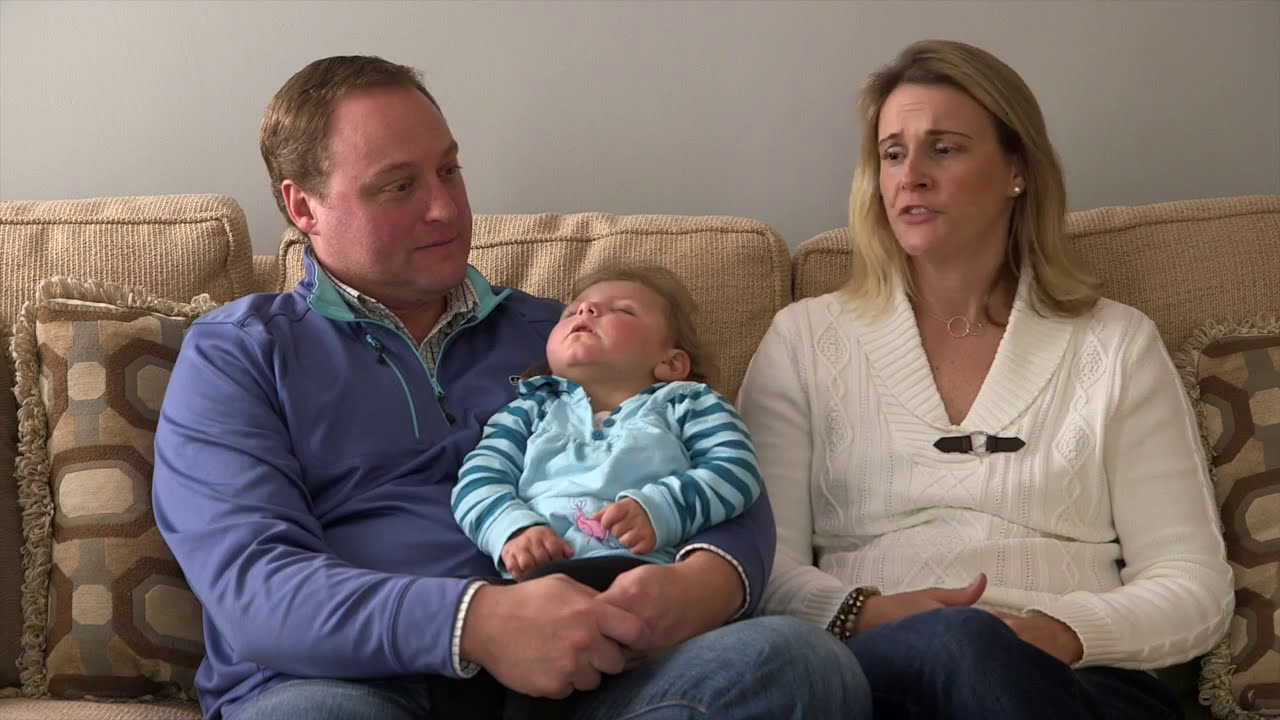In this photograph, a family of three is seated on a brown sofa with patterned cushions, against a light gray wall. On the left, an adult man, possibly in his 30s or 40s, holds a sleeping baby on his lap. The man, who has short brown hair, is wearing a blue-colored jacket over a white checkered button-down shirt and light blue jeans. His gaze is directed slightly downward and to the right, towards the baby. The baby, dressed in green and blue striped clothes, rests with its head back, deeply asleep. To the right of the man, a woman with shoulder-length blonde hair sits, seemingly mid-conversation with her mouth partially open. She is wearing a white sweater, blue pants, pearl earrings, a gold necklace with a hoop pendant, and two bracelets on her right wrist. The scene captures a serene and intimate family moment.